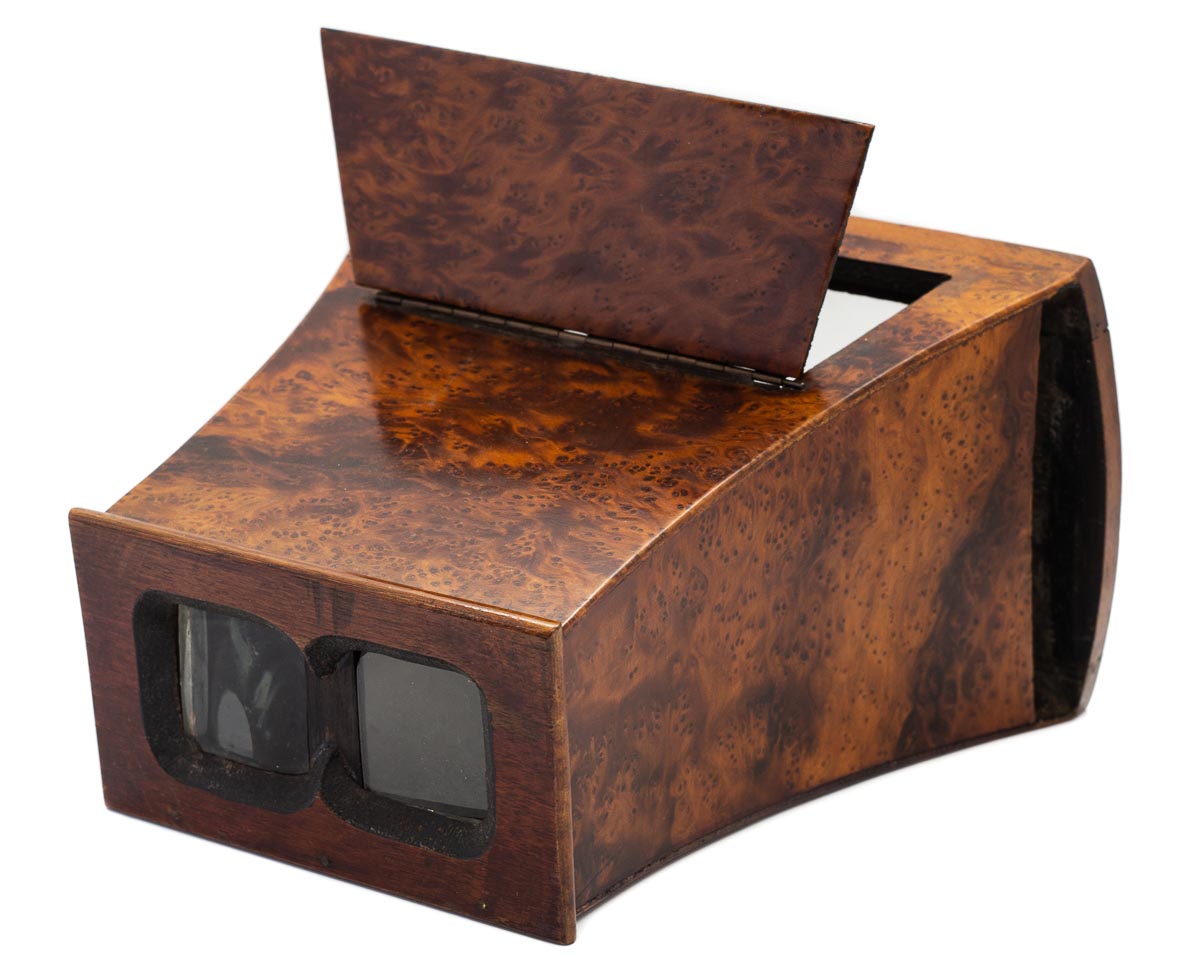The image depicts a color photograph of an antique, wooden viewfinder, reminiscent of a pair of binoculars. The medium-brown wood, complemented by spots of black, gives it a distinctly aged appearance. The device features a flap at the top that flips open and appears to serve an unspecified purpose. The front of the viewfinder is notable for its two small square lenses, set within two larger square frames, which seem designed for the user to look through. These lenses likely allow the viewer to see a photograph inserted into the device. The entire object is isolated against a completely white background, with no other visible supports or surroundings.